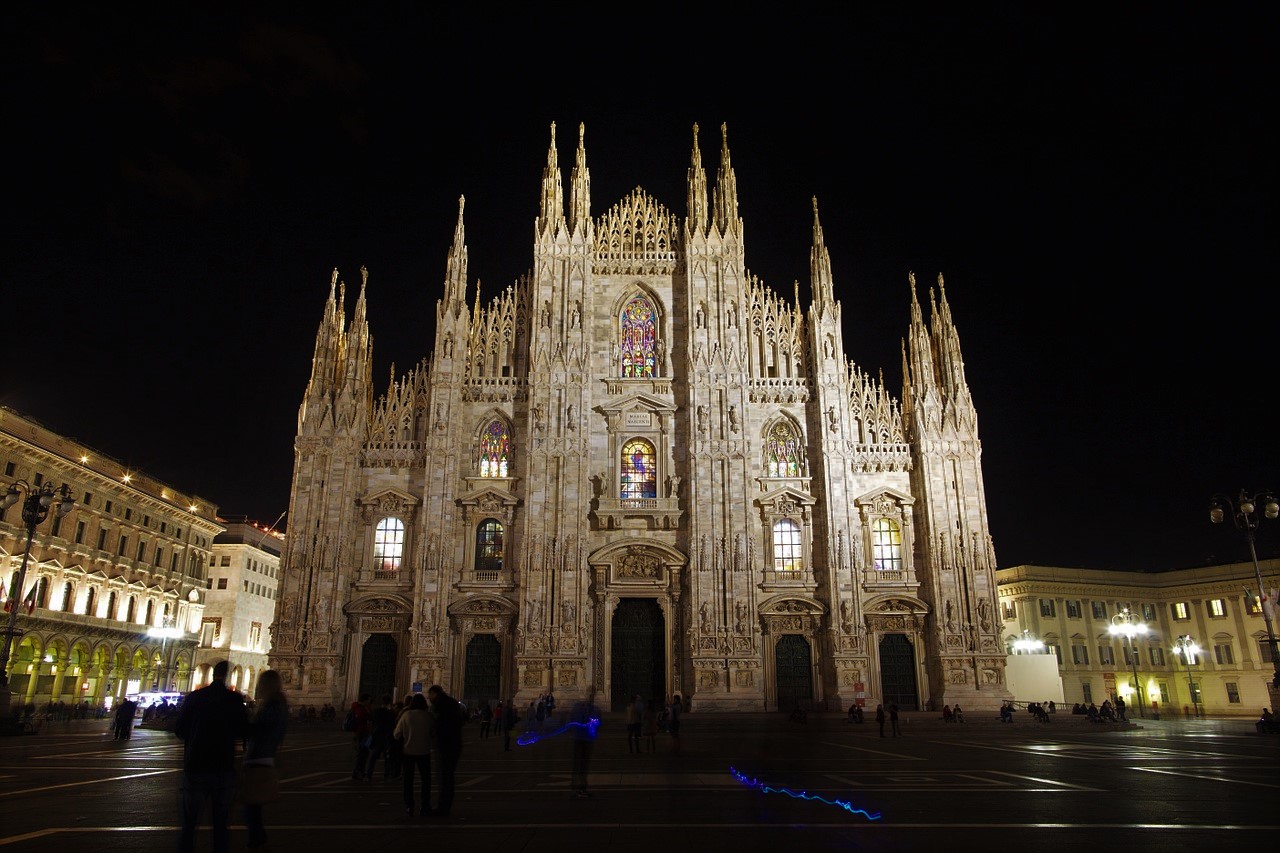This nighttime photograph depicts a historic gothic-style cathedral, most likely situated in a European plaza or courtyard. The cathedral serves as the focal point of the image, characterized by its intricate stonework and a triangular facade that reaches upward, flanked by six progressively taller spires adorned with intricate carvings, giving its exterior a detailed, almost "wrinkly" appearance. The cathedral boasts five grand doorways; the central door is the largest, with two on each side. Above these doors are several stained glass windows in vivid hues of red, blue, green, white, and yellow, casting a colorful glow.

Surrounding the cathedral, there's a public square paved with what appears to be wet concrete or dark ground, where the dim outlines of people can be seen, some stopping to take photographs, indicating its popularity as a tourist destination. The adjacent buildings are illuminated with their lights on, contrasting against the pitch-black sky. These structures, likely from the Napoleonic or Baroque era, are lower in height, about three to four stories tall, horizontally arranged, and punctuated by warm, glowing windows that frame the cathedral. Altogether, this composition creates an evocative scene of historical architecture against a serene nighttime backdrop, capturing the serene yet grand essence of the space.